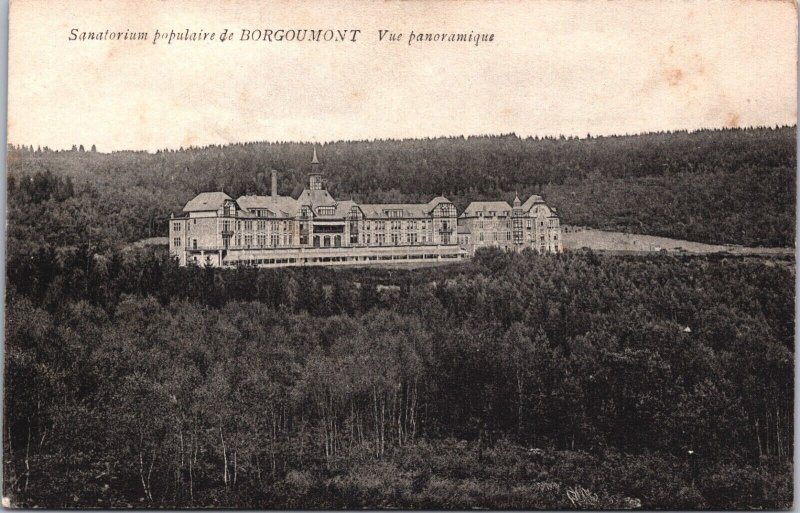This is a black-and-white photograph, possibly a sepia-toned postcard, depicting the expansive Borgermont Sanatorium, identified by the French text 'Sanatorium Populaire de Bourgemont Voupanouramique' at the top. The image showcases a very large, Victorian-style stone building, with a distinct sharp steeple in the center, situated atop a hill and surrounded by a vast expanse of dense trees. The immense structure, likely spanning four to five stories, features an impressive facade with approximately 30 windows. The sky in the image appears to have a slightly pinkish hue, suggesting a daytime setting. The sanatorium's remote, forested location emphasizes its isolation and grandeur.